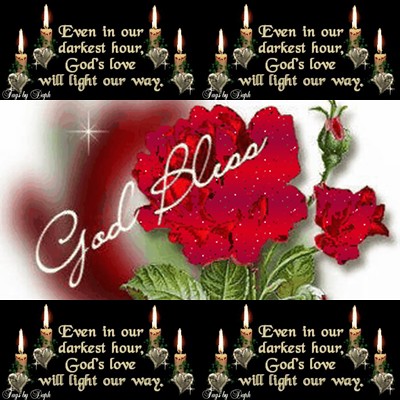The image features a detailed and vibrant red rose as its centerpiece, situated against a dark backdrop. The rose has one prominently open bloom accented by delicate green leaves, a smaller rose off to the lower right, and a tiny rosebud positioned slightly above it on the right side. Overlaid diagonally across the open rose, the words "God Bless" are elegantly written in white cursive.

The photograph is framed by thick black panels both at the top and bottom, each adorned with several lit candles that cast a warm, gentle glow. These panels feature a repeated comforting message in white cursive: "Even in our darkest hour, God's love will light our way," written twice side-by-side. Centered at the bottom, beneath this repeated phrase, the word "Thank you" appears discreetly and elegantly in small cursive letters. Some glitter on the rose adds a subtle shimmering effect, enhancing its beauty and the overall emotional impact of the image.